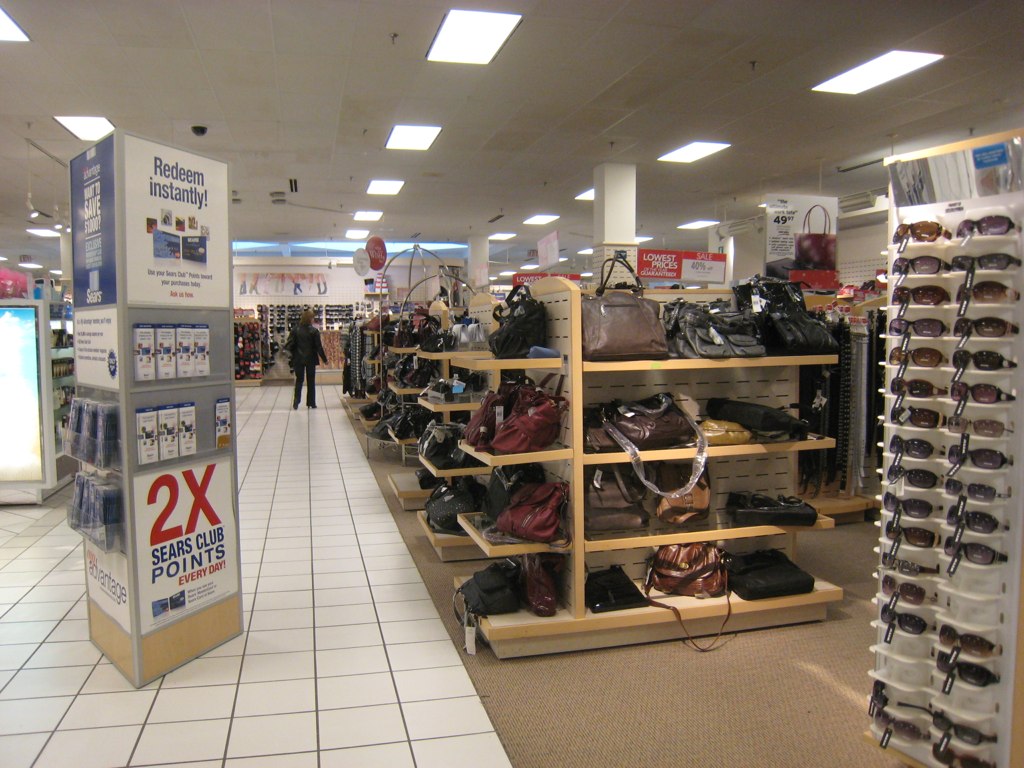This indoor color photograph, taken inside a Sears department store, showcases a well-lit shopping environment with distinct sections and clear signage. On the right side of the image, there are multiple brown-colored displays, each housing four shelves of handbags in various shades of brown, black, burgundy, and tan. Adjacent to this is a tall, white, plastic sunglasses rack featuring two vertical columns, each holding about 20 pairs of sunglasses in assorted shades, primarily brown and black. 

Prominently placed in the foreground is a rectangular, approximately two-meter-tall sign with various promotional information. The top part of the sign announces "Remedy Instantly," followed by a section with brochures, and below it, the text "2X Sears Club Points Every Day" in large red and blue letters. This sign is positioned on a white-tiled floor that extends throughout the main walkway, while the areas featuring products are carpeted.

The ceiling, which is visible in the background, is adorned with white tiles and rows of fluorescent rectangular lights. To the left of the main display, another price sign is noticeable, characterized by its red rectangular shape with white lettering proclaiming "Lowest Prices" and "Sale 40% Off." A lone shopper is seen in the distance with their back turned, adding a sense of scale and activity to the scene.